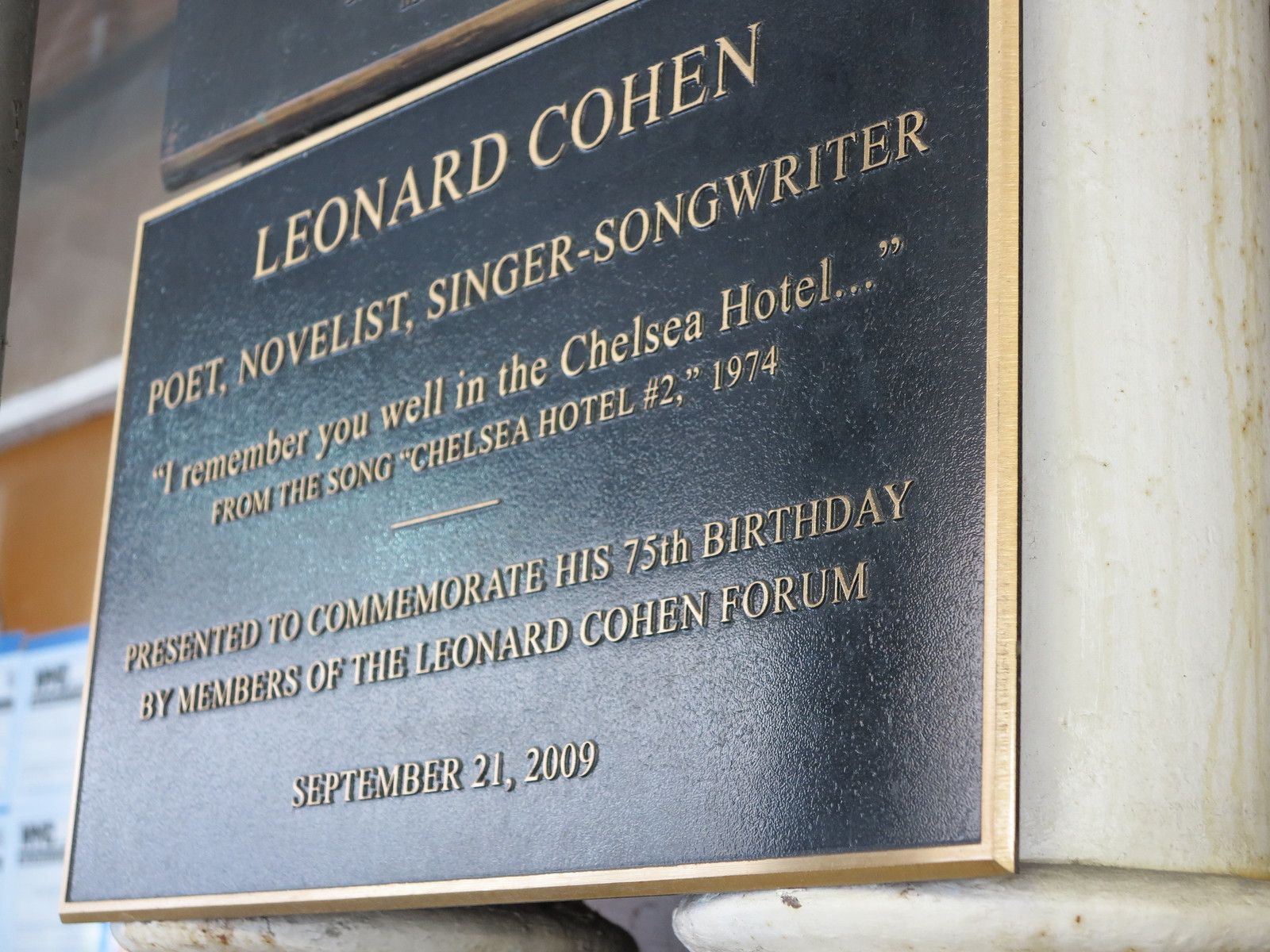The image features a shiny, reflective black plaque with a gold rim, mounted on an exterior wall with various patterns and colors. Above the plaque, part of another plaque is visible. The inscription on the black plaque, written in yellowish-gold font, reads: "Leonard Cohen, Poet, Novelist, Singer-Songwriter." Below this, a quote from Cohen's song is inscribed: "I remember you well in the Chelsea Hotel... from the song Chelsea Hotel No. 2, 1974." Further down, a small dash precedes the text, "Presented to commemorate his 75th birthday by members of the Leonard Cohen Forum." At the bottom, the date "September 21, 2009" is listed. The plaque is set against a wall, possibly at a corner, contributing to its distinct visual presence.